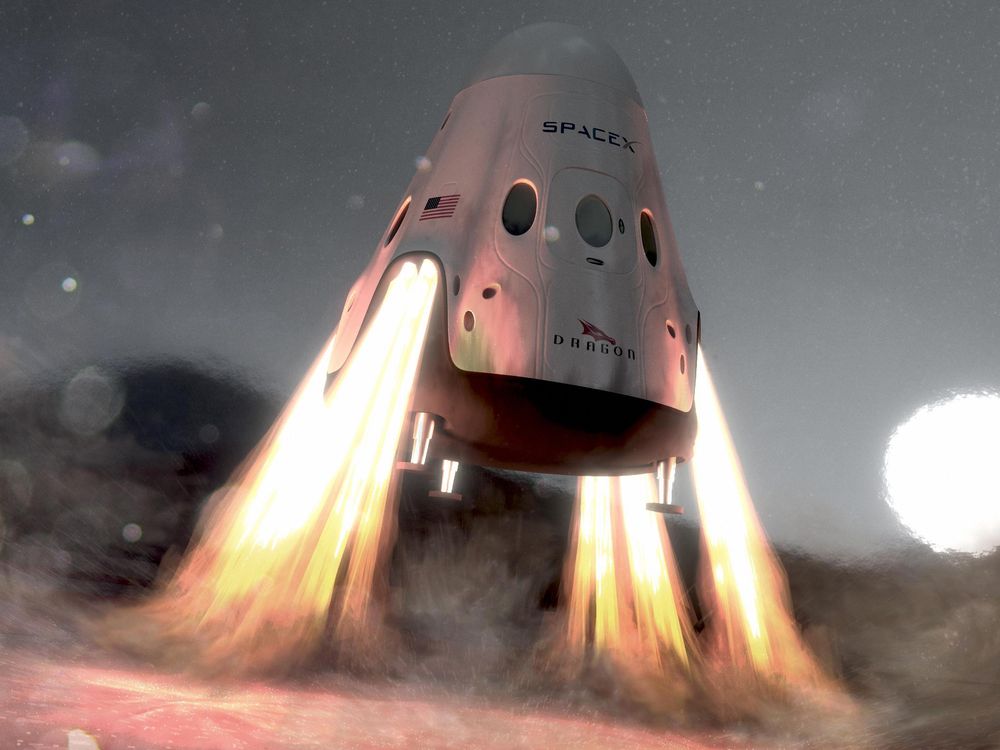The image depicts a computer-animated SpaceX spacecraft named Dragon, in the midst of takeoff or landing. The spacecraft has a sleek, silver metallic body with a rounded dome top and a gradual, angling shape towards the bottom. On the front, the words "SpaceX" are prominently displayed, accompanied by an American flag to the left and the word "Dragon" with a small dragon logo towards the bottom. There are three oval windows along the side and additional oval details prominent on the front. The craft is supported by three silver legs ending in brown, flat, rounded pads. Flames and orange and yellow projections are visible beneath the spacecraft, emitting from under its edges. The background is gray and slightly blurred with a faint cloud pattern, emphasizing a circular beam of light on the bottom right, which could be a depiction of a sun, moon, or another planet. The ground beneath is indistinct but suggests the outline of hills or a small hill, adding depth to the scene. Several smaller moons or celestial bodies are subtly scattered throughout the sky.